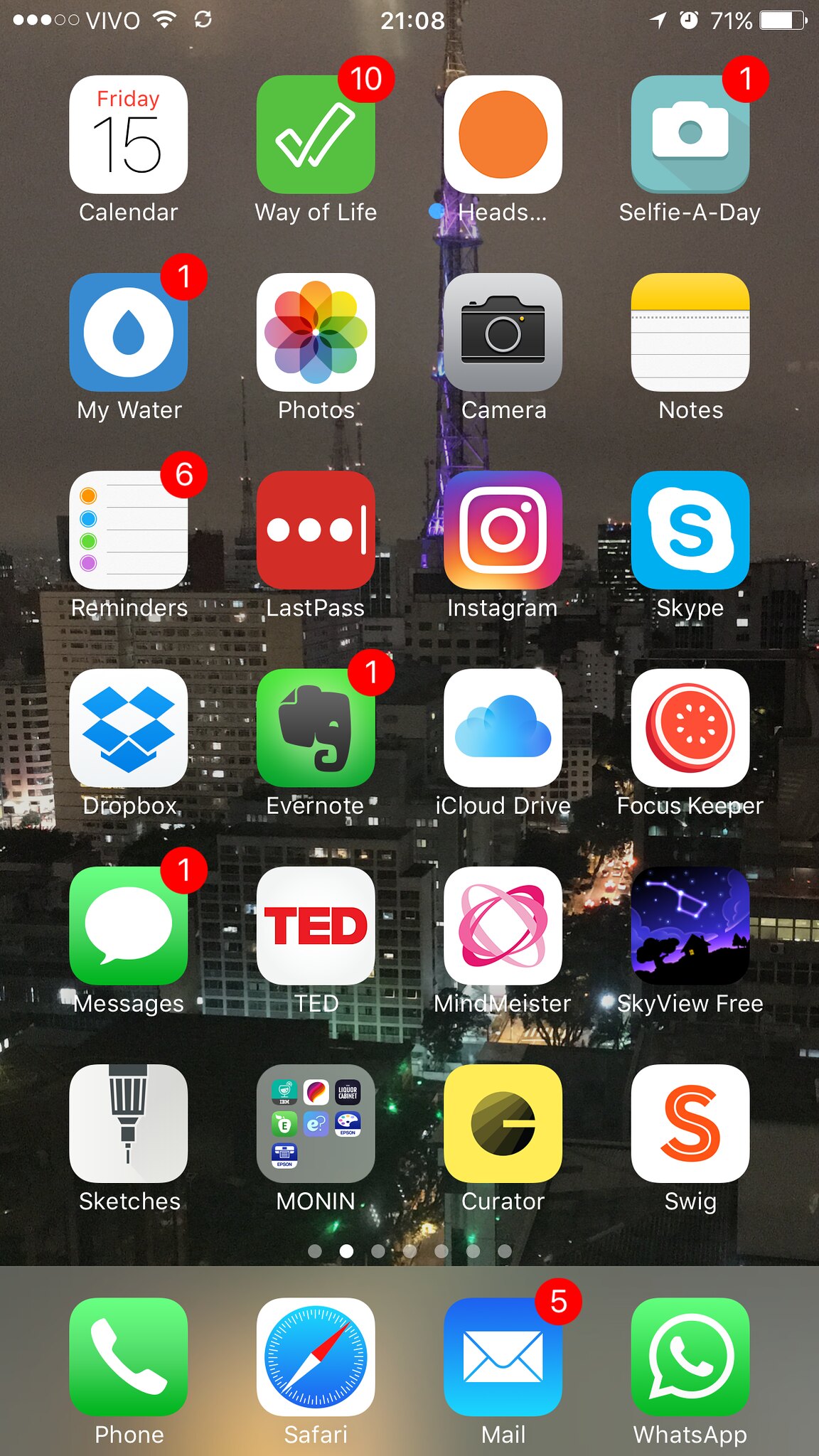This image is a screenshot of the home page of a smartphone. The home screen displays a grid of application icons arranged in four columns and six rows. Additionally, there is a seventh row at the bottom with a light gray shaded background that contains four square icons for essential apps: Phone, Safari, Mail, and WhatsApp.

The wallpaper is a stunning image of a city skyline at night, featuring numerous multi-story high-rise buildings with illuminated windows. Dominating the scene is a tall communications tower, lit with striking purple and white lights, standing prominently above the other structures. Other tall building spires are visible in the background, adding to the urban panorama.

At the top of the screen, the brand name "Vivo" (V-I-V-O) is displayed. Adjacent to it are various status indicators: the Wi-Fi signal icon, the refresh icon, and the battery level, which is currently at 71%. The time shown on the device is 21:08.